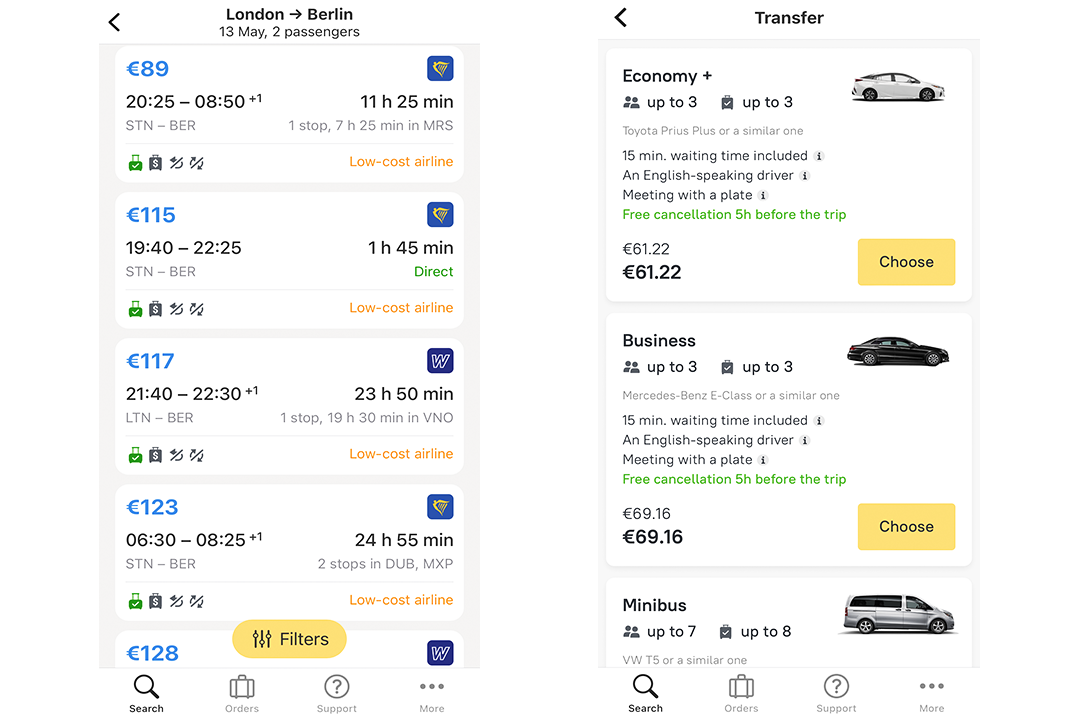The image consists of two vertically rectangular screenshots displayed side by side within a slightly horizontally rectangular frame, depicting a likely car rental interface. 

### Left Image:
- **Header**: "London to Berlin, 13th of May, two passengers"
- **Content**: Contains several vertical listings
  - Each listing includes:
    - **Time**: Depicting travel duration
    - **Details**: Noted as "low-cost airline," but more fittingly representing car travel times
- **Footer**: Features icons for "Search," "Orders," "Support," and "More"

### Right Image:
- **Header**: "Transfer" (top center)
- **Content**: Displayed vehicle options, including:
  - **First Listing**: "Economy Plus, Up to 3" with an image of a hatchback
  - **Second Listing**: "Business, Up to 3" with an image of a sedan
  - **Third Listing**: Partially visible, "Minibus" with an image of a minivan

The detailed presentation suggests a digital platform for booking car rentals, highlighting travel specifics, and a selection of vehicle categories.